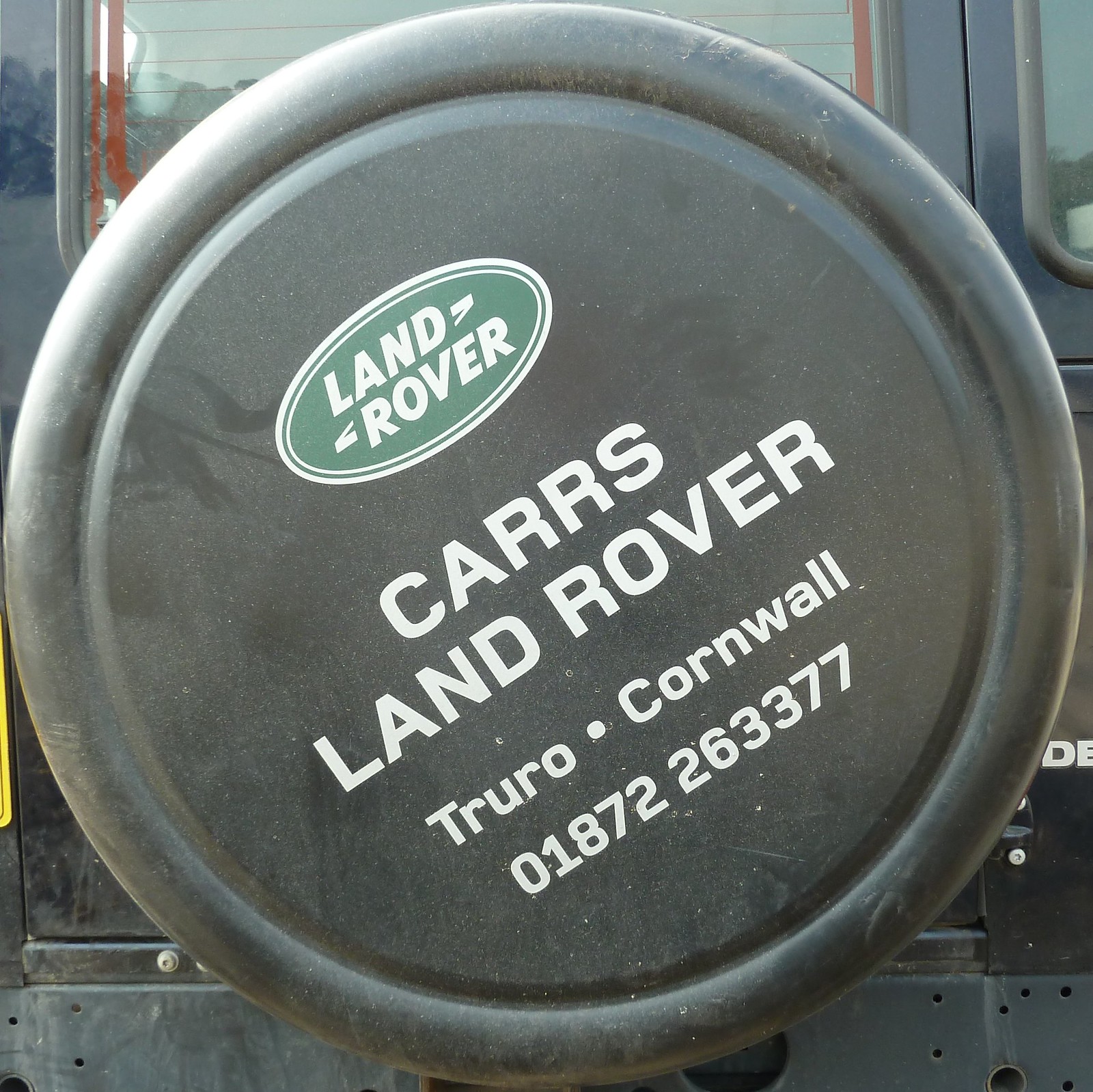This photograph captures a close-up view of the rear of a black Land Rover vehicle, focusing on the spare wheel cover centrally positioned in the image. The wheel cover is a prominent black circle adorned with the distinctive green Land Rover logo and the text "Land Rover" in white font. Below, it reads "Cars, Land Rover, Truro, Cornwall" along with the phone number "01872-263377". Surrounding the wheel cover, the black metal frame of the vehicle is visible, along with the rear window that features orange defrosting lines. The setting appears to be outdoors in daylight, providing a well-lit, detailed perspective of the Land Rover's rear end.